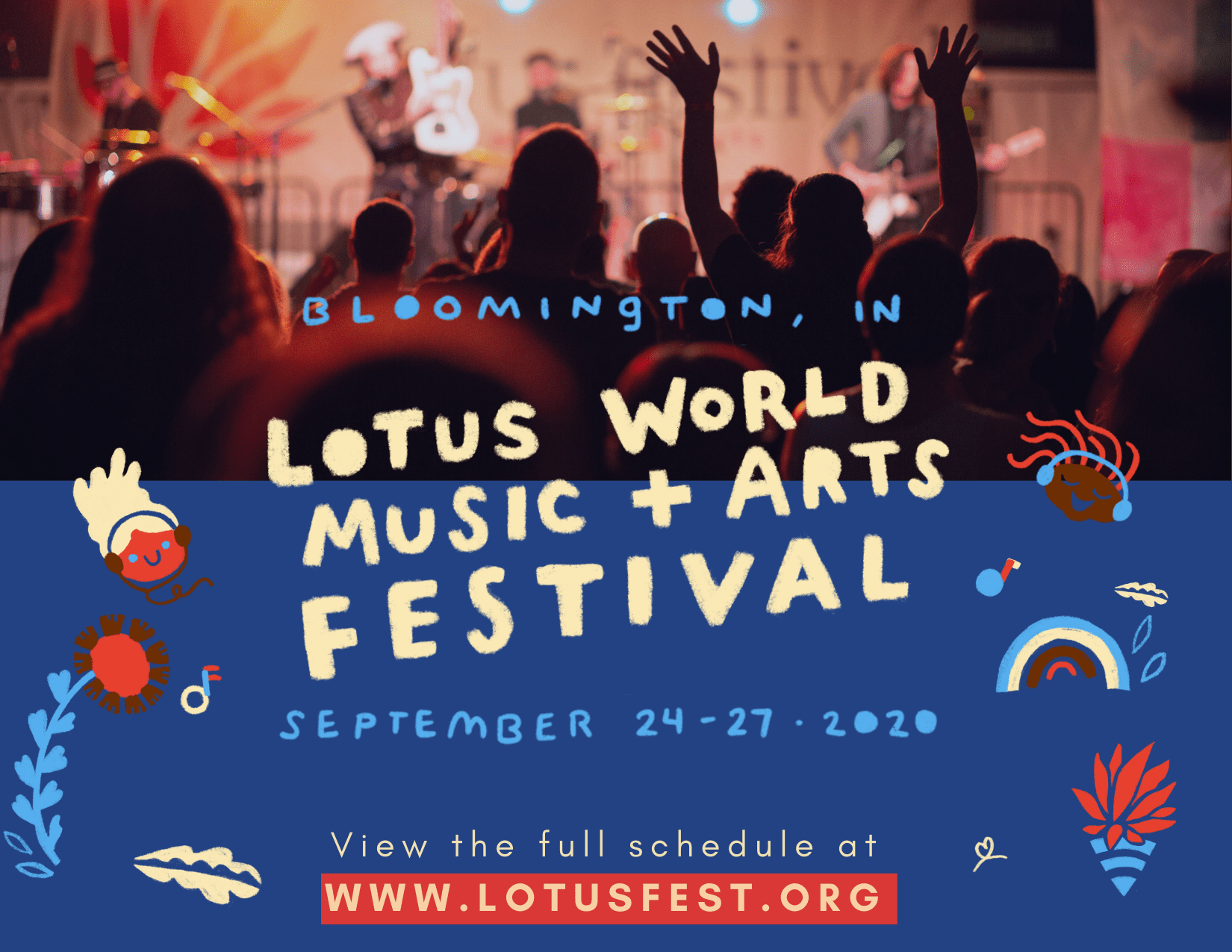The advertisement for the Lotus World Music and Arts Festival captures the vibrant and lively atmosphere of the event. The top half of the image features a photograph of a crowd, their faces full of excitement, standing in front of a stage where musicians with guitars are performing energetically. The stage is slightly blurred, emphasizing the dynamic nature of the performance. One person in the crowd is seen with their hands raised, adding to the sense of enthusiasm.

The bottom half of the background is a solid dark blue, providing contrast and focus to the text and artwork above. Over the photograph, in bold blue text, the location "Bloomington, Indiana" is prominently displayed. Just below it, the festival's name, "Lotus World Music and Arts Festival," is written in eye-catching yellow text.

Further down, dates "September 24th through 27th, 2020" appear in blue, providing essential details for potential attendees. Completing the informational portion, the phrase "View the full schedule at www.lotusfest.org" is shown in yellow, guiding viewers to more details.

Enhancing the playful and artistic vibe of the advertisement, various drawn and animated images surround the text. Among these are a colorful flower and a vibrant rainbow, symbolizing the festival’s creative diversity. Musical notes float around, indicating the musical focus of the event. On either side of the central text, two drawn faces are depicted—one with orange-ish colored skin and the other with black skin—both wearing headphones, symbolizing the universal love for music and the inclusive nature of the festival.